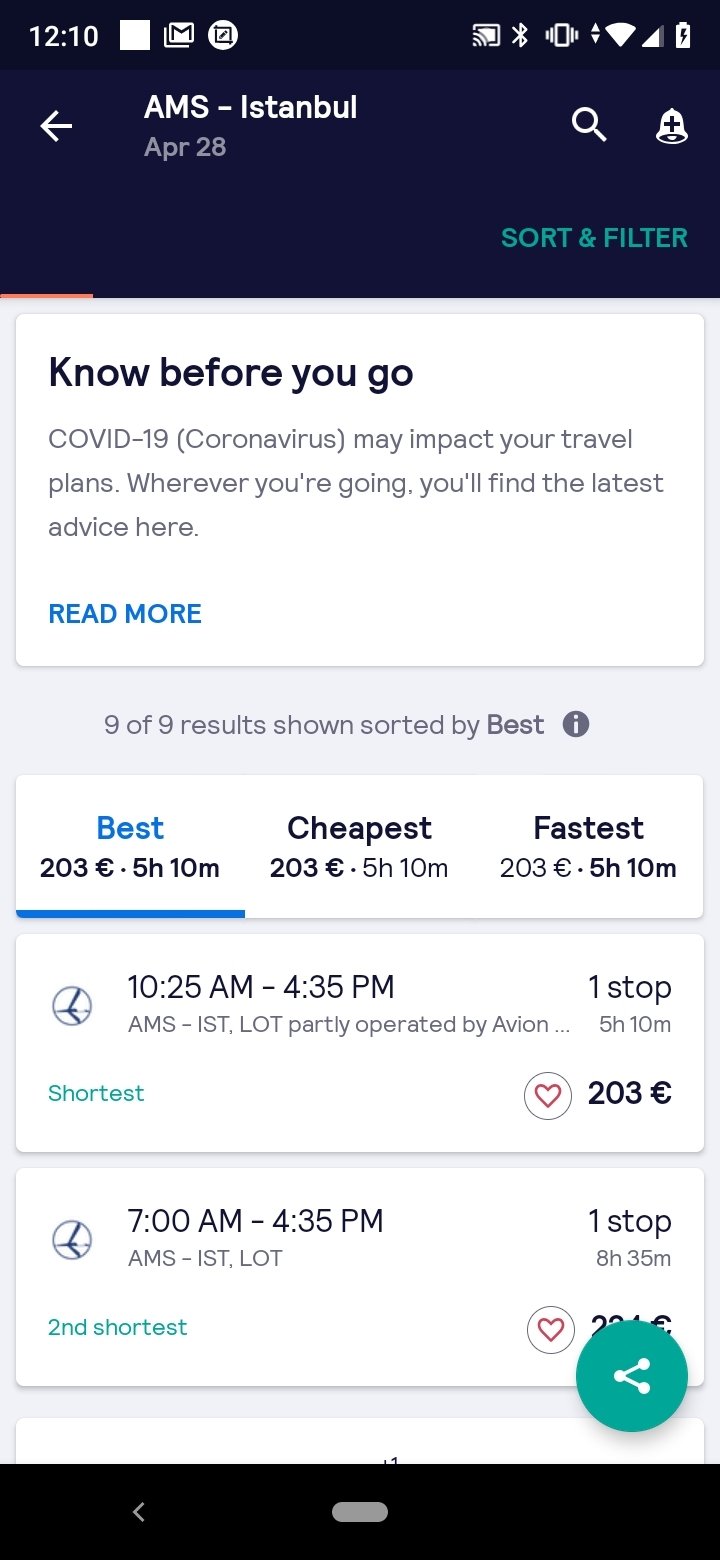Screenshot of an Android phone displaying a travel-related app.

At the top, a black horizontal bar contains several icons, including a magnifying glass and a bell with a plus sign, indicating search and notification functionalities. Below this, the screen shows a travel booking section with an entry labeled "AMS - Istanbul."

The date "APR 28" is prominently displayed, suggesting a travel schedule. The screen also features sorting and filtering options. The main content area is divided into several sections. One section is labeled "Know Before You Go," highlighting important COVID-19 information with a prompt to read more for the latest updates.

The app indicates that 9 out of 9 results are shown, sorted by "Best." An information icon ("i" within a circle) is also displayed. Below this, the screen lists various travel options with prices starting at €203 and estimated travel durations like "5h 10m."

A specific listing notes a partially operated flight by "Avalon" with a "5h 10m" duration and a "One Stop" detail. 

In the lower right corner, there's a share icon represented by a teal triangle with lines connecting its corners, pointing to a sharing functionality. The overall design features light gray backgrounds and intuitive layout for ease of use.